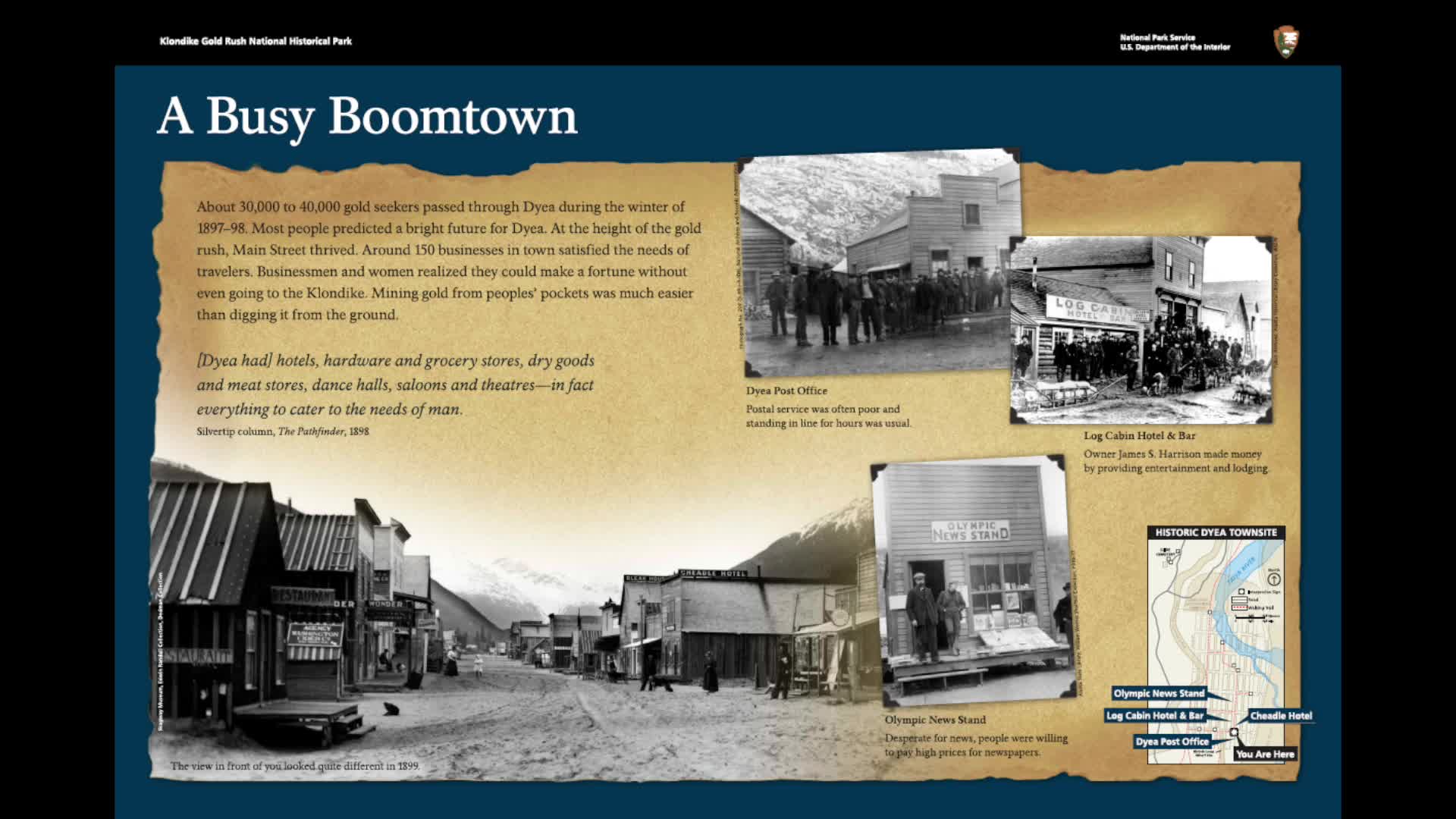This informational slide, originating from the National Park Service, features a detailed depiction of Dyes, a bustling boomtown during the gold rush era of 1897-1898. The slide is framed with a dark blue border and titled "A Busy Boomtown" in white letters at the top. The central section of the slide mimics aged, torn paper in brownish-yellow tones, adding a historical touch. 

The central text reveals that between 30,000 to 40,000 gold seekers passed through Dyes during the winter of 1897-98, and the town flourished with around 150 businesses catering to travelers' needs. The narrative highlights Main Street's vibrant, thriving atmosphere, predicting a bright future for Dyes during the height of the gold rush.

The imagery includes several historical photographs placed around the text. One key picture, located at the bottom center of the slide, shows an old town with wooden buildings lining a dirt road, reminiscent of the cowboy era. Additional photographs on the right capture moments from the town's bustling past, including gatherings of townspeople. In the bottom-right corner, a map details various significant sites referred to in the text above. This comprehensive visual and textual presentation immerses viewers in the rich history of Dyes as a pivotal gold rush hub.